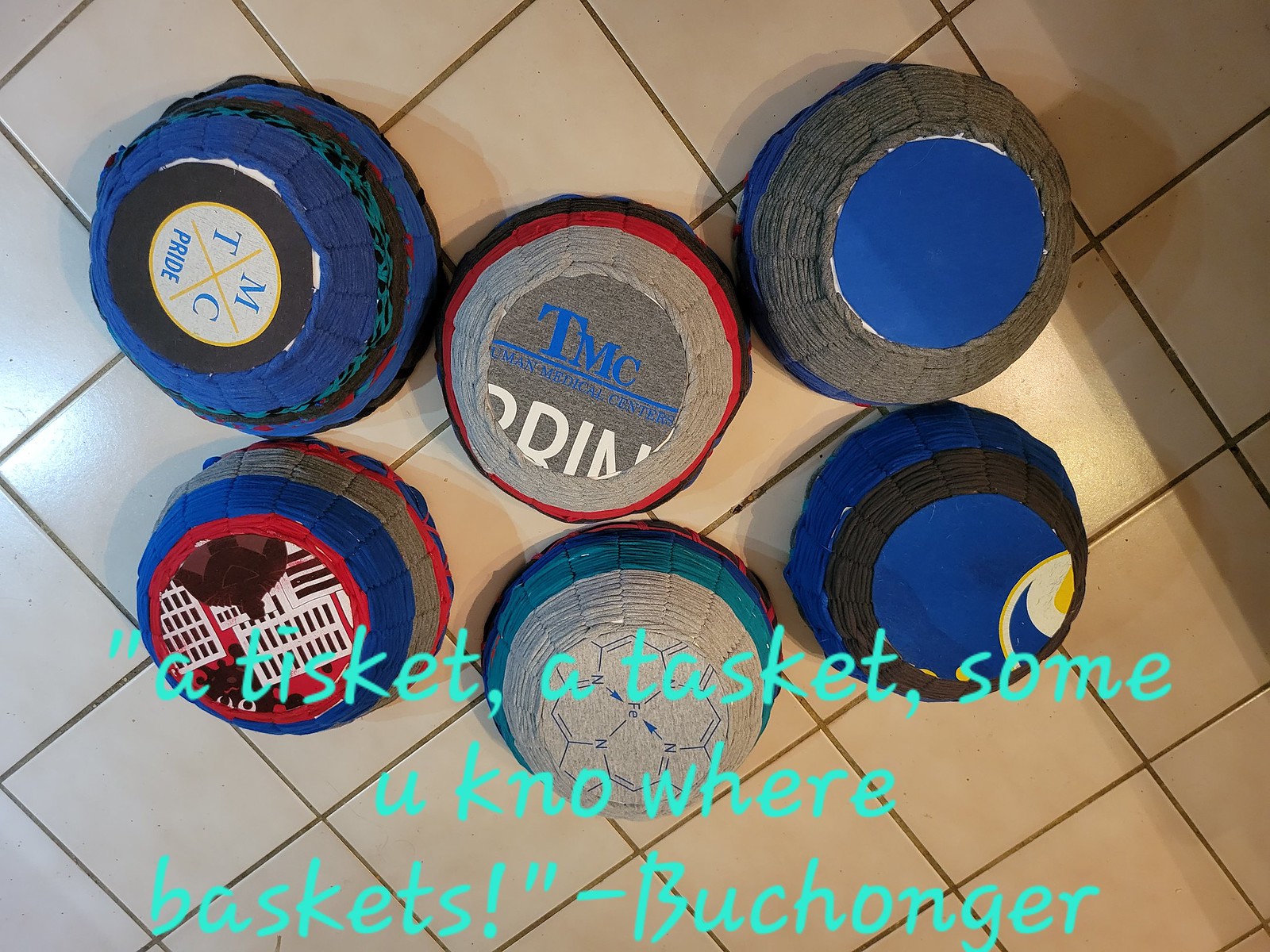The photograph captures six homemade baskets, all flipped upside down to showcase their bottoms. Each basket is intricately woven from fabric, including repurposed t-shirt material, and features a variety of emblems such as a cartoony Godzilla scene, a chemical formula, university logos, and sports team references. Predominantly in shades of blue, black, red, and gray, these colorful baskets rest on a white tile floor with dark brown grout. Text overlaid on the image reads, "A-tisket, a-tasket, some you know wear baskets," attributed to Buchonger. The image appears to be promotional, possibly from an Etsy page, advertising customizable baskets crafted from t-shirts and woven fabric.